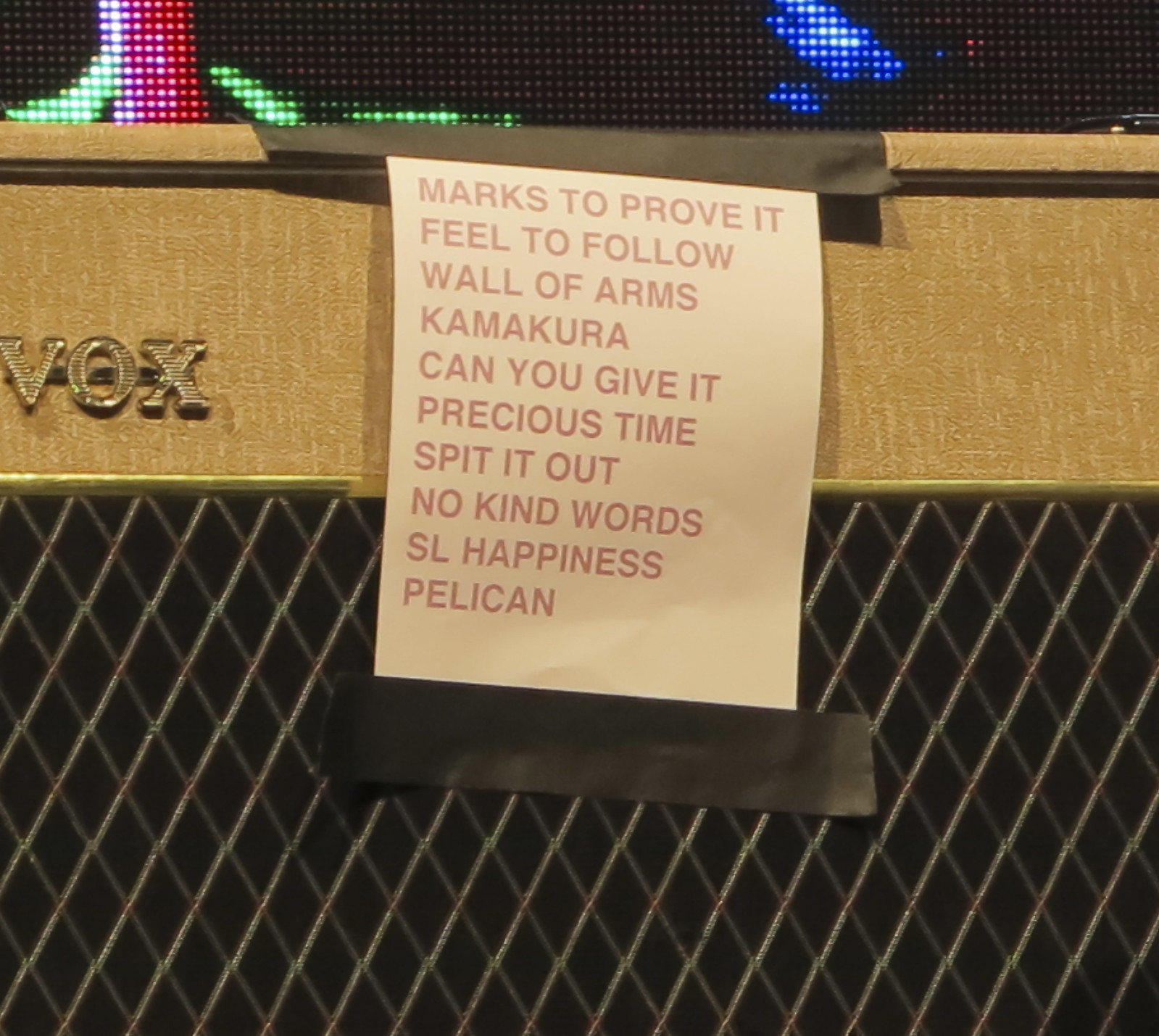The image features a white sign with red, all-caps text randomly listing phrases such as “marks to prove it,” “feel to follow,” “wall of arms,” “Kamakura,” “can you give it precious time,” “spit it out,” “no kind words,” “S.L. happiness,” and “Pelican.” This sign is taped at the top and bottom with black electrical tape to what seems to be a golden-brown boombox with silver wiring. On the left-hand corner of the boombox, part of the name is visible, reading “V.O.X.” The sign itself partially covers a metal backboard with a crisscross, diamond-shaped pattern. Above this setup, there appears to be a pixelated image, reminiscent of a Lite-Brite, with visible red, green, and blue dots forming a colored pattern.